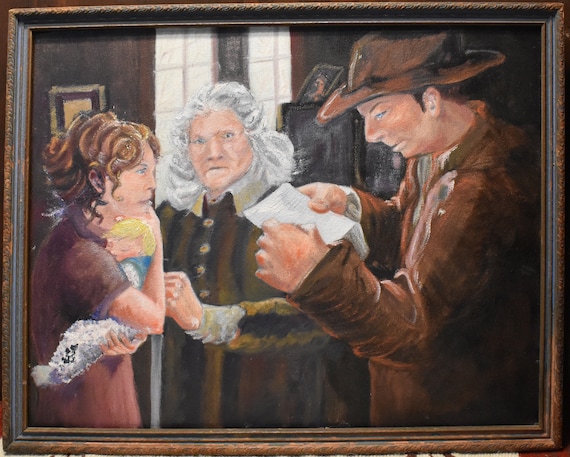The image is a detailed, color photograph of an oil painting, housed in a wooden frame. The rectangular painting, displayed horizontally, depicts a scene with three Caucasian individuals and a baby, all indoors. On the left, a younger woman with curly, dark reddish-brown hair is dressed in a dark reddish shirt and holds a baby wrapped in a blue blanket, close to her chest. The baby has golden blonde hair and appears to be asleep. Centrally positioned, an older man with white, long, and slightly floofy hair wears an elegant brown coat with lacy sleeves, reminiscent of colonial attire. He appears slightly confused and gazes towards the paper being held by a man on the right. This man is portrayed as an inspector or detective figure, dressed in a brown trench coat and matching hat. He has blue eyes and is intently reading from a piece of paper. Behind them, a white window indicates their indoor setting.